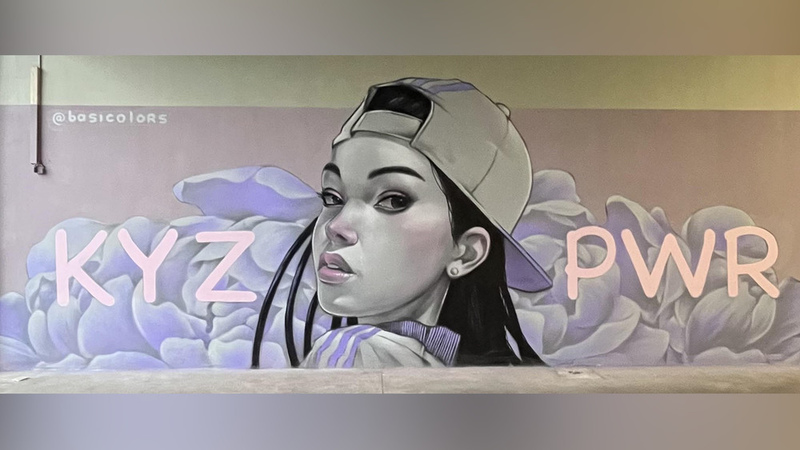This image portrays an intricately detailed street mural showcasing a girl with black hair, wearing a backwards baseball cap adorned with purple stripes that blend into her skin tone. Her facial features are meticulously rendered, showing expressive black eyebrows, intense black eyes, pink lips, and rosy cheeks with a hint of a pinkish nose. She sports a purple and white shirt, and a white studded earring is visible as she turns her head to engage the viewer directly with a captivating stare. 

The mural is set against a predominantly purple background that gradates to a lighter shade on the left side. Prominent capital letters "K-Y-Z" are painted in white on the left side of the mural, while "P-W-R" appears in whitish-pink letters on the right. At the very top left corner, there is a tag labeled @BASICOLORS (spelled B-A-S-I-C-O-L-O-R-S), indicating the artist's handle. The overall composition of the mural is framed by a purple border, with a yellowish-white banner accentuating the top section.